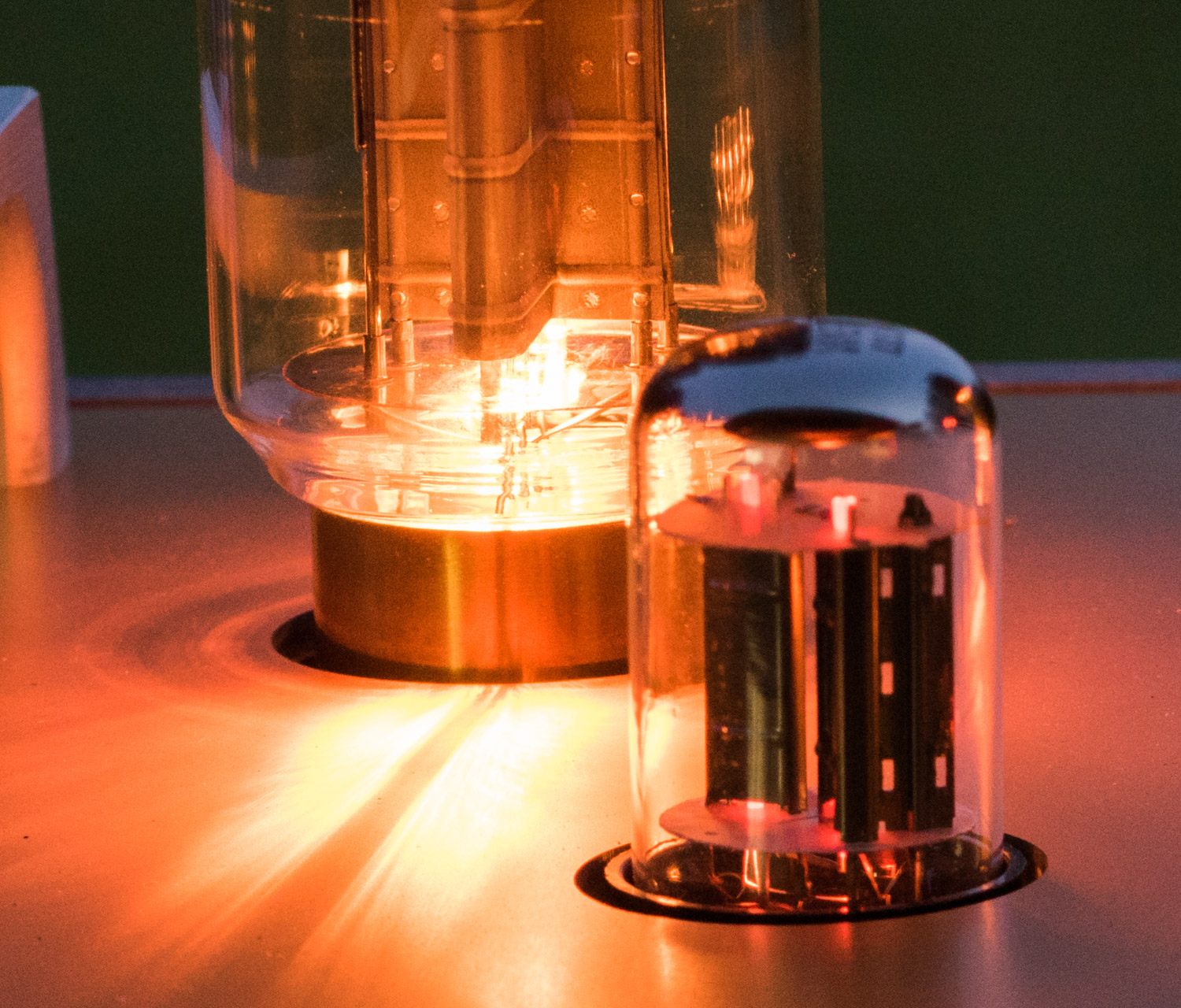The image depicts a dark setting featuring two glass domes mounted on a metal surface, potentially part of laboratory equipment or a steampunk-themed machine. The smaller dome is positioned in the foreground and contains a structure emitting a faint red glow, reminiscent of buildings. This structure appears black and has metallic elements standing upright inside it. To the center-left, the larger dome is partially visible and illuminated from beneath with a warm golden-yellow light. This dome, featuring metallic elements, is mounted on a base that resembles golden hinges under clear glass. The overall aesthetic is industrial, with elements of stainless steel, and the two glass domes vary in size, with the larger one in the background and the smaller one in the foreground, both contributing to a mysterious, almost mechanical scene.